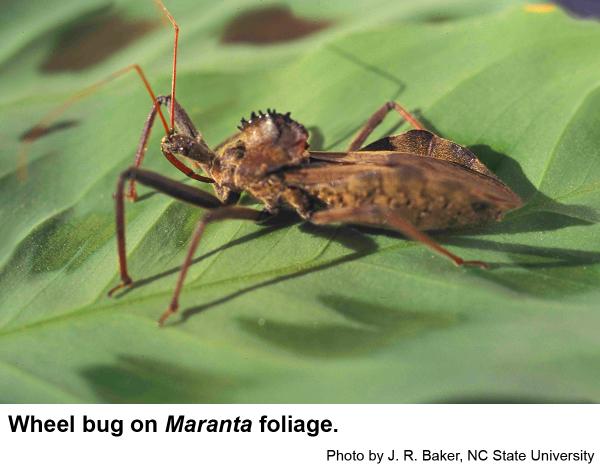The image showcases a detailed, close-up view of a brown Wheel Bug resting on a large, green Maranta leaf, which entirely fills the background like a soft, veined blanket. The insect's body is light brown with darker brown shades, and it has a cigar-shaped form. Its head, adorned with small notches, features long, thin, orange-brown antennae extending forward. The Wheel Bug appears motionless, its segmented legs planted firmly on the leaf's surface. The bug’s carapace includes a distinct hump on its back, adorned with sharp, black spikes, and what looks like a small cape over its body. The photograph is credited at the bottom: "Wheel Bug on Maranta Foliage. Photo by J.R. Baker, NC State University."